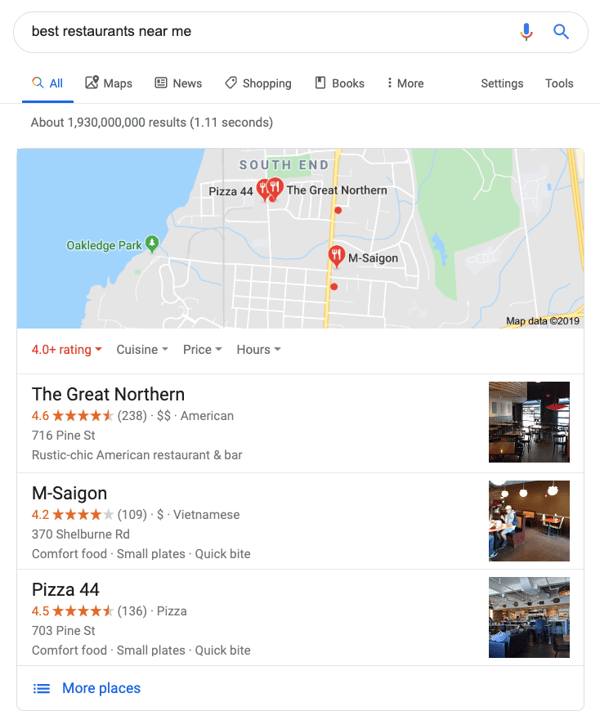A detailed screenshot of a search for "best restaurants near me." At the top, the search bar displays the query. Navigation options are visible: "All," "Maps," "News," "Shopping," "Books," "More," "Settings," and "Tools." Below, a map highlights various restaurant locations. Just beneath the map, filters for "4.0+ ratings," "Cuisine," "Price," and "Hours" are available. 

The list features three restaurants:

1. **The Great Northern**
   - **Rating:** 4.6 stars (238 ratings)
   - **Price Range:** $$
   - **Cuisine:** American
   - **Address:** 716 Pine Street
   - **Type:** Rustic Chick, American Restaurant and Bar
   - **Image:** Exterior view of the restaurant.
   
2. **M-Saigon**
   - **Rating:** 4.2 stars (109 reviews)
   - **Price Range:** $
   - **Cuisine:** Vietnamese
   - **Address:** 370 Shelbourne Road
   - **Type:** Comfort Food, Small Plates, Quick Bite
   - **Image:** Interior view showing brown walls and flooring, with a person sitting at a bar and a couple of tables in sight.
   
3. **Pizza 44**
   - **Rating:** 4.5 stars (136 reviews)
   - **Cuisine:** Pizza
   - **Address:** 703 Pine Street
   - **Type:** Comfort Food, Small Plates, Quick Bites
   - **Image:** Interior view with a white ceiling and dark flooring, limited visibility of other features.
   
At the bottom, an option to see "More Places" is available.